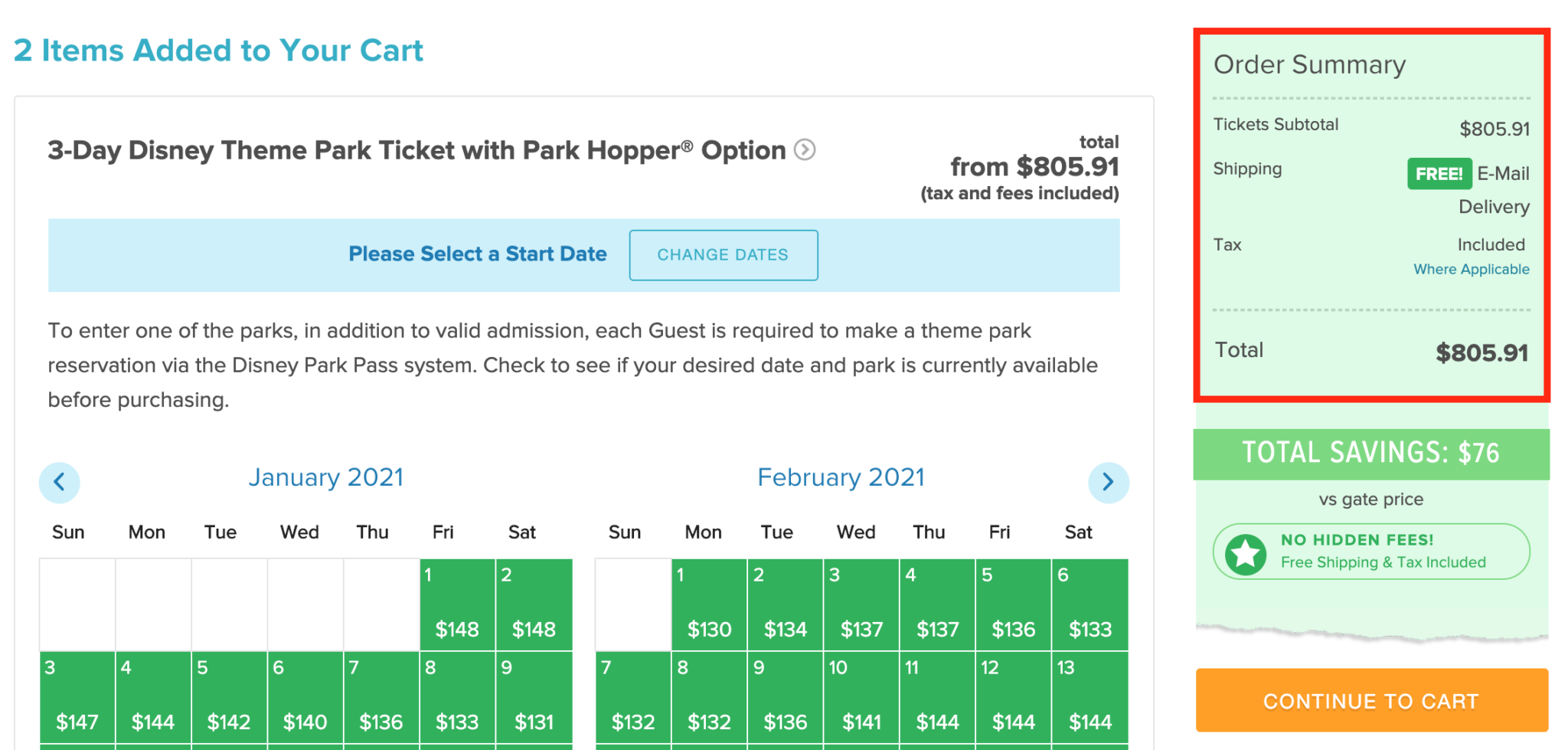Displayed against a pristine white background, a green banner at the top indicates that two items have been added to your cart. The items include a Three-Day Disney Theme Park Ticket with Park Hopper option, totaling $805.90 (tax and fees included). Below the total, a blue rectangle prompts you to "Please Select a Start Date."

Next to it, another blue rectangle allows you to "Change Dates." Important information follows, stating that in addition to valid admission, each guest is required to make a theme park reservation via the Disney Park Pass system. It advises you to check if your desired date and park are currently available before purchasing.

Two calendars showcase the first two rows of January 2021 and February 2021. January dates start on Friday, the 1st, and end on Saturday, the 9th. February dates begin with Monday, the 1st, and extend to Saturday, the 13th, each day displaying corresponding prices.

An order summary is outlined in red, listing a ticket subtotal of $805.90, with free email delivery for shipping, including applicable taxes. The final total remains $805.90.